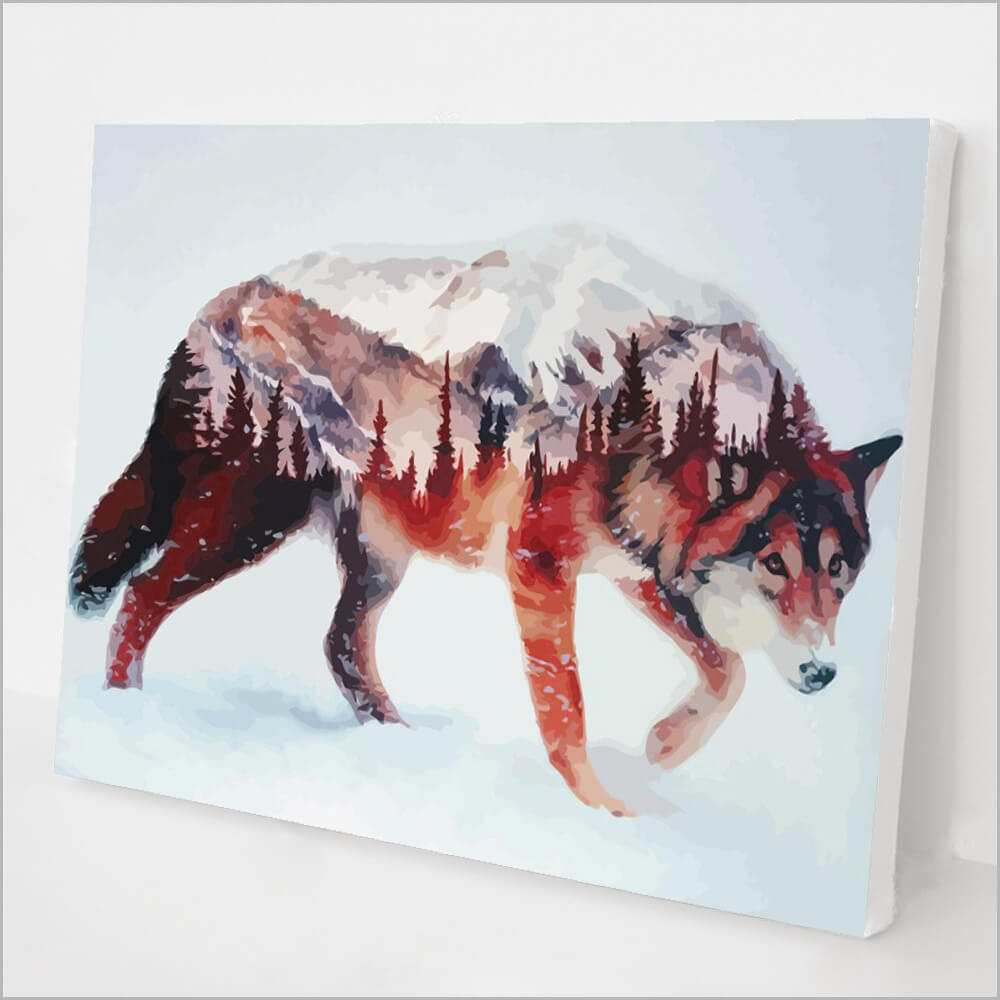In the image, we see a serene painting leaning against a creamy, off-white wall. The large canvas captures a tranquil snowy landscape at the bottom transitioning seamlessly into a light blue sky. Dominating the composition is a striking wolf, depicted in a unique mosaic-like style with a mix of colors such as brown, dark brown, black, red, and orange. The wolf's posture suggests movement as it walks forward, head slightly bowed into the snow. Intriguingly, the body of the wolf incorporates another image—a detailed portrayal of a mountainous scene with snow-capped peaks and tall pine trees rising prominently, creating the illusion that its body is composed of these natural elements. This layered depiction not only highlights the natural beauty of the snowy environment but also brings a mystical quality to the wolf, integrating its form into the landscape it inhabits.